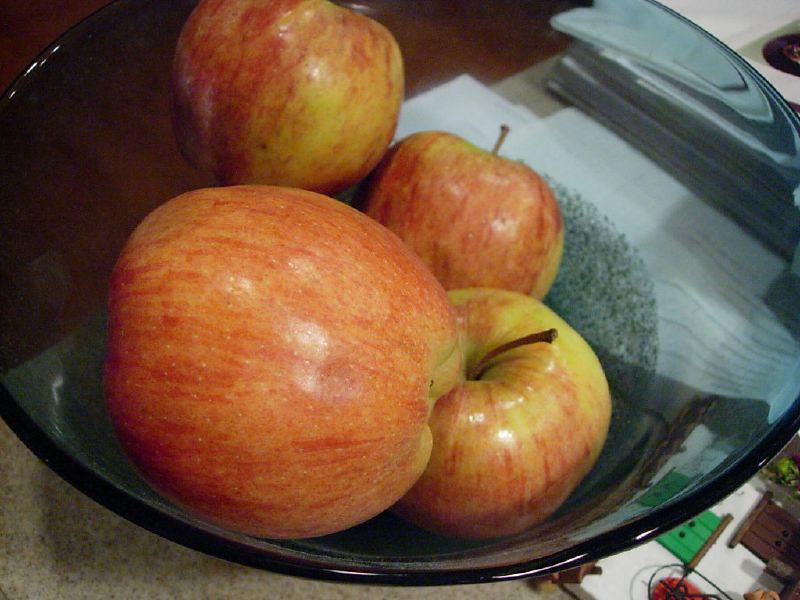A detailed indoor color close-up photograph captures a round glass bowl with a slight blue tint, containing four fresh apples. The apples are positioned predominantly to the left of center. Two apples rest at the bottom of the bowl with their tops and stems visible, while the other two are stacked to the left and on top of them. The apple in the foreground on the left lies on its side, showing its bottom rather than the stem. 

In the upper left corner of the image, there's a dark area lacking details. The lower left corner features what seems to be a tan paper or placemat beneath the bowl. Through the glass bowl, which is transparent, the upper right corner reveals a stack of paperwork. The lower right corner displays a patterned item, likely depicting bird feeders, possibly on a notepad or tablecloth.

The apples, exhibiting a blend of orangish and greenish hues, appear fresh with no blemishes or insect damage. The photograph is well-lit and in sharp focus, highlighting the subtle reflections of light on the apples' surfaces. No text or print is visible in the image.